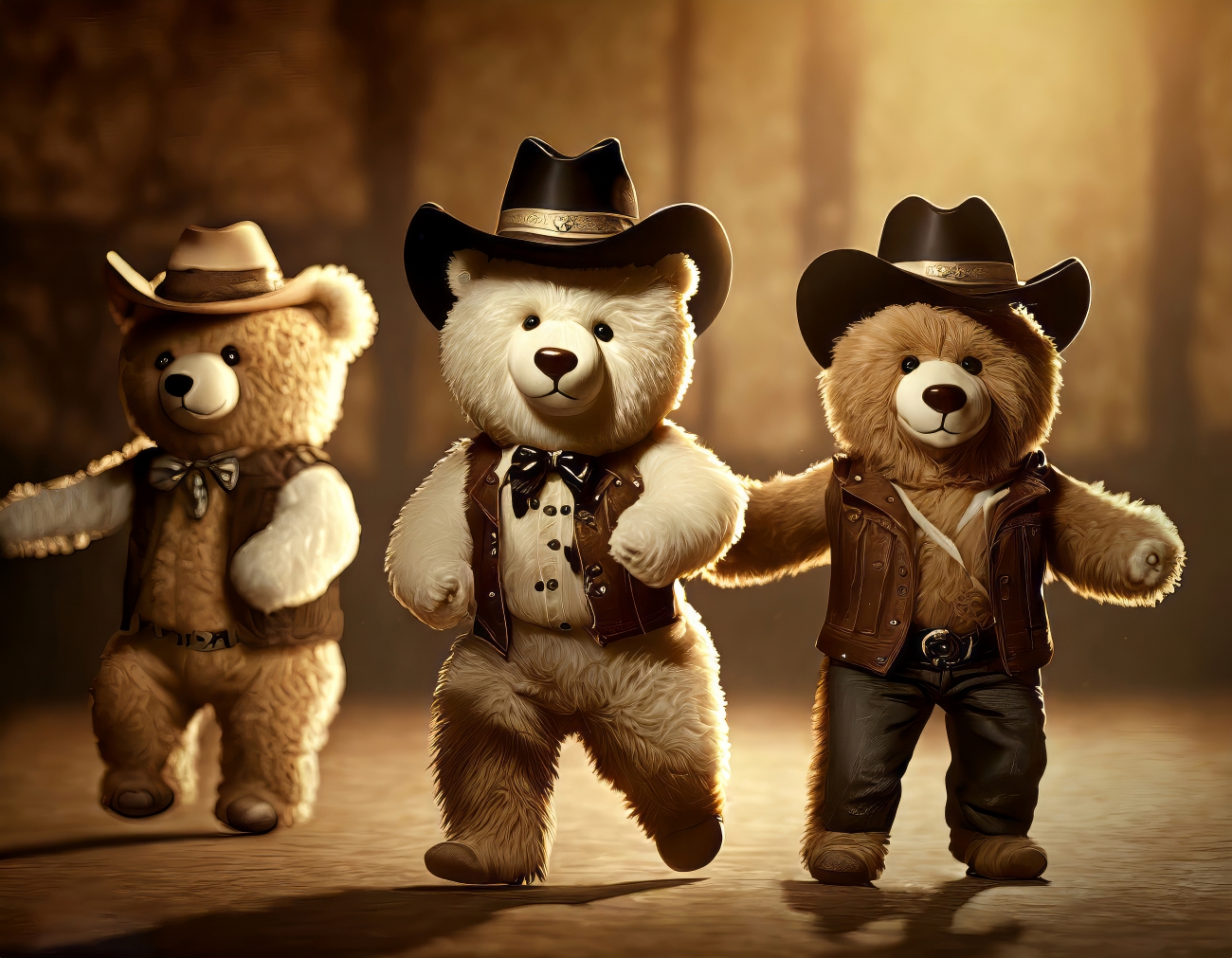This charming image showcases three stuffed teddy bears dressed in cowboy attire, walking towards the camera. Each bear sports a cowboy hat adorned with bronze or gold-toned bands. The teddy bear on the far right has a tan cowboy hat, a matching tan vest, blue jeans with fringe along the outside edge, and a prominent belt buckle. The middle teddy bear, lighter in color, wears a vest and a bow tie with a shirt underneath, evidenced by visible buttons, but no pants. The left teddy bear, similar in tan color to the right bear, dons a brown cowboy hat with a darker trim, a brown vest, a black and white bow tie, and a fancy belt. They are positioned on a brown floor against a brownish background, with the rightmost bear standing still while the other two appear to be in mid-step, giving a sense of movement. The image has an amber-colored filter, adding a warm, nostalgic feel to the scene.